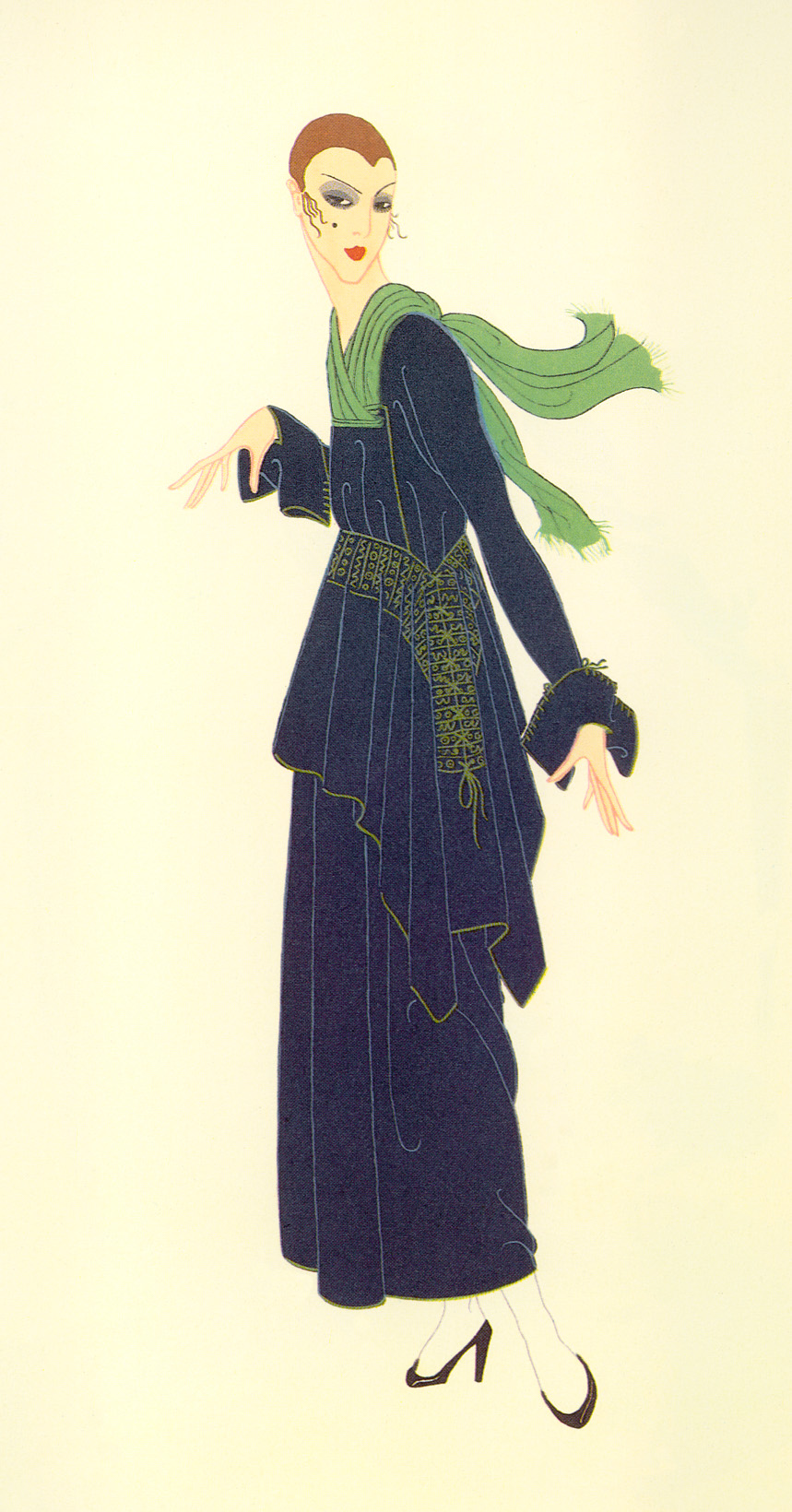The image depicts a detailed, elegant painting of a Caucasian woman standing in a side profile pose, her body twisted slightly to gaze at the viewer. She is wearing a dark blue, long-sleeved dress with intricate greenish-gold and yellow fringe detailing around the waist and vertical stitching running through the fabric. A light green scarf is draped elegantly around her neck, cascading down her back, forming a collar-like appearance. The woman's legs are pale, almost white, accentuating her black high-heeled shoes. Her brown hair is styled back with some curls framing her face, which is adorned with red lipstick and a mix of blue and gray eyeliner. The background of the painting is a solid off-white color, providing a stark contrast that highlights the woman's poised and graceful figure, centered vertically in the rectangular frame, twice as tall as it is wide.